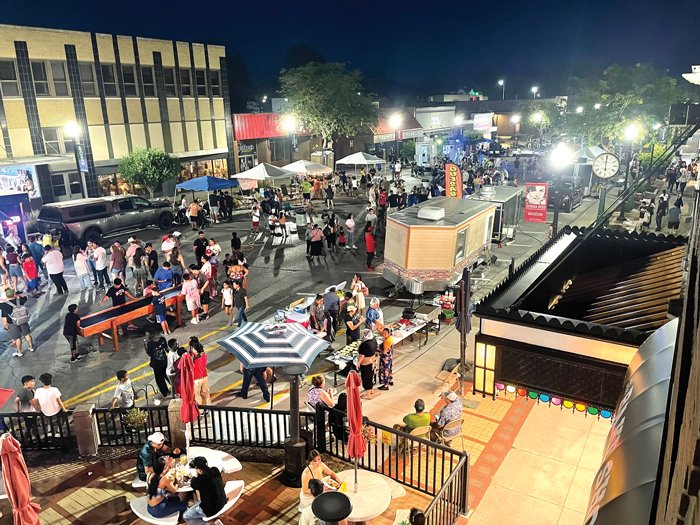This nighttime photograph captures a vibrant street scene in a bustling city, illuminated by an array of streetlights casting a warm glow over the area. The dark blue, almost black sky creates a striking backdrop for the lively festivities below, resembling a block party or a bustling night market. Scattered throughout the streets are numerous stands; some trailers serve as food vendors, while others offer clothing, knickknacks, and merchandise. People are seen enjoying the atmosphere, standing around chatting, or sitting at tables enjoying their meals. Towards the center-left, a table with a black top appears to be set up for a game, drawing a small crowd. In the top right corner, between two streetlights, an analog clock stands prominently, its hour and minute hands both pointed at 12, although its distance makes it slightly hard to discern. The entire scene exudes a sense of community and enjoyment, with everyone seemingly having a wonderful time under the night sky.